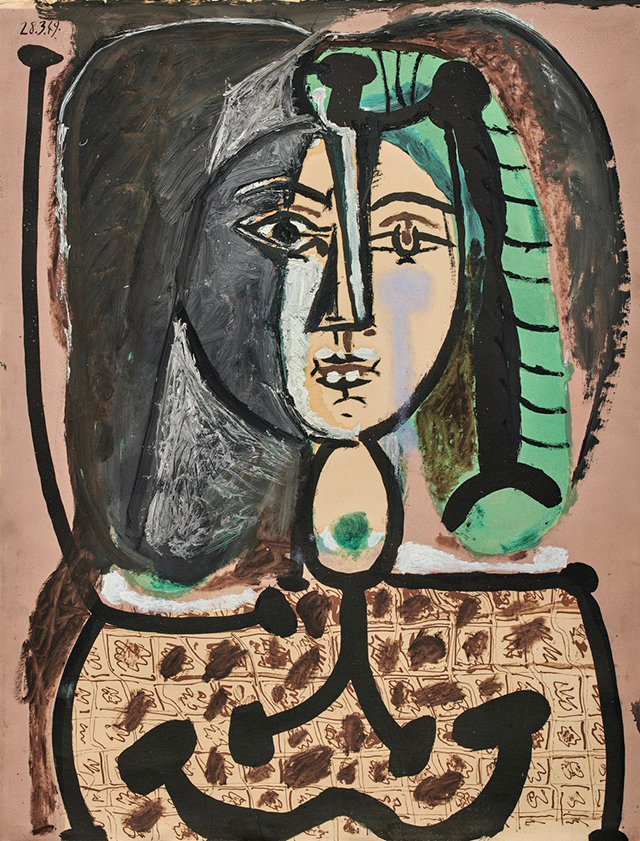This is a color lithograph in portrait orientation by Picasso, rendered in a cubist style. The subject is an abstract representation of a woman’s face. The depiction is asymmetrical, with the face featuring dark brown eyebrows and mismatched eyes; the left eye is more detailed with a white sclera surrounding a dark brown iris, while the right eye is less defined and only sketched. Her nose is triangular, with dark, alternating black and white stripes projecting downward from the forehead. The complexion splits into two differing tones; the right side is lighter tan, whereas the left side is painted in grayscale tones with some black areas. Her hair is greenish-aqua on the right and absent on the left, with a gray shadow replacing it.

A distinct head covering evokes an Egyptian or mummy-like appearance. There's a mixture of geometric shapes and abstract patterns throughout the body, described as being elliptical in shape but disproportionately small compared to the head, with stick-like legs extending outwards, each ending in rudimentary feet. The body is adorned with a black, upside-down V-shape detailing, a squiggly line, and patterned squares with brown dots. The background varies with brown tones interspersed with some green on the right side and black on the left, contributing to the overall abstract composition.